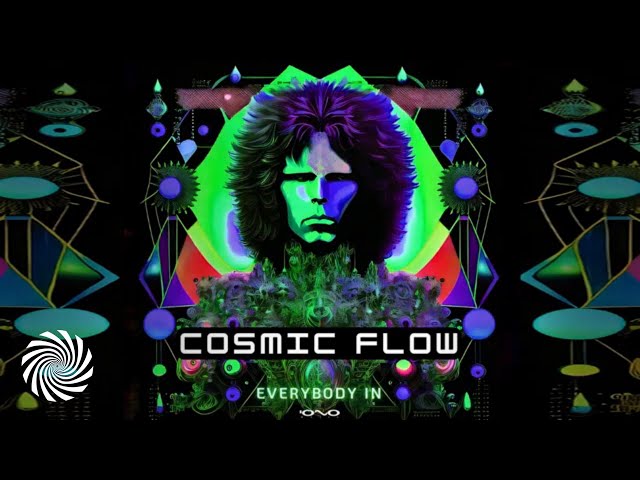The image appears to be a psychedelic digital album cover with a striking black background. Dominating the center is a stylized drawing of a man resembling David Bowie, with long, flowy 1970s hair illuminated by neon green, black light purple, and lavender purple lights. His green skin is divided into lime green, indigo blue, and lilac purple hues, with his eyes obscured by shadows from his brow. Surrounding his face are 3D, swirling, and geometric designs, including turquoise circles and gold lines on both sides, connected by triangles. In the bottom left corner, there's a hypnotic black-and-white spiral. In front of the man, white text reads "Cosmic Flow," followed by "Everybody In" in neon green. Overall, the image exudes a vibrant and geometrically intricate psychedelic art style.